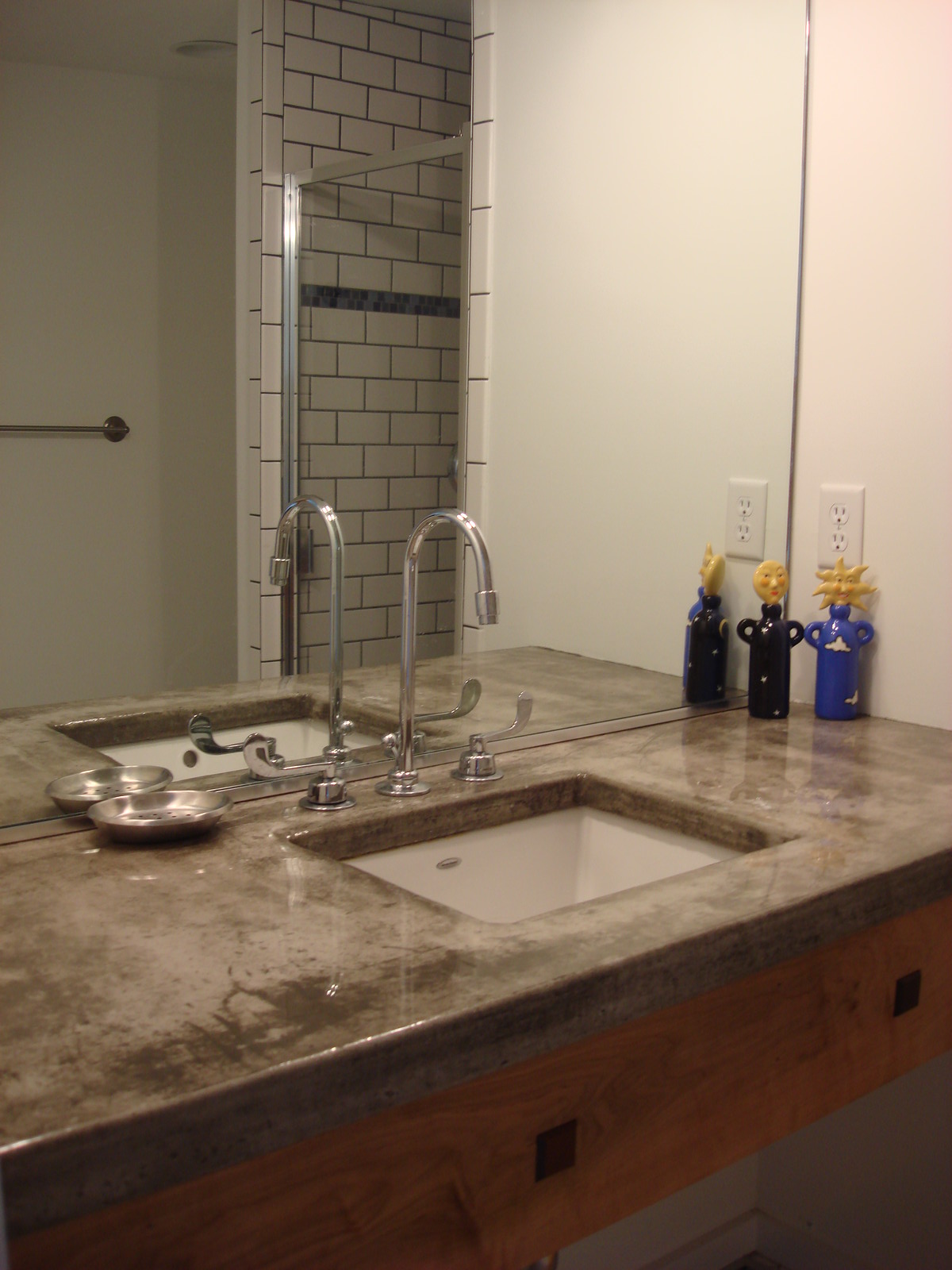The image captures a well-appointed bathroom, centered on a large rectangular mirror reflecting the shower and towel rack. The countertop extends from the left to the right, predominantly on the left side, featuring a deep, white sink embedded in a gray marble surface with shades of gray and brown, appearing as if covered by a subtle white cast. Below the counter, a medium brown wood grain cabinet with two black handles provides a structured border that does not extend to the floor. The bathroom walls are white, while the floor remains out of view but suggests a cream-colored tone.

A sleek, silver faucet with high arching curves and two swooping handles sits above the sink. On the countertop, two decorative bottles with yellow tops shaped like shells or stars stand out; a black bottle with two looped handles on the left, and a similar blue bottle on the right. An empty, silver soap tray, round and resembling a shell, is placed to the left of the sink. 

In the mirror's reflection, an empty dark silver towel rack is visible. Adjacent to it, the shower boasts a glass door and a striking black and white tile design, accented by a horizontal black border running through the center, completing the luxurious and tasteful bathroom scene.